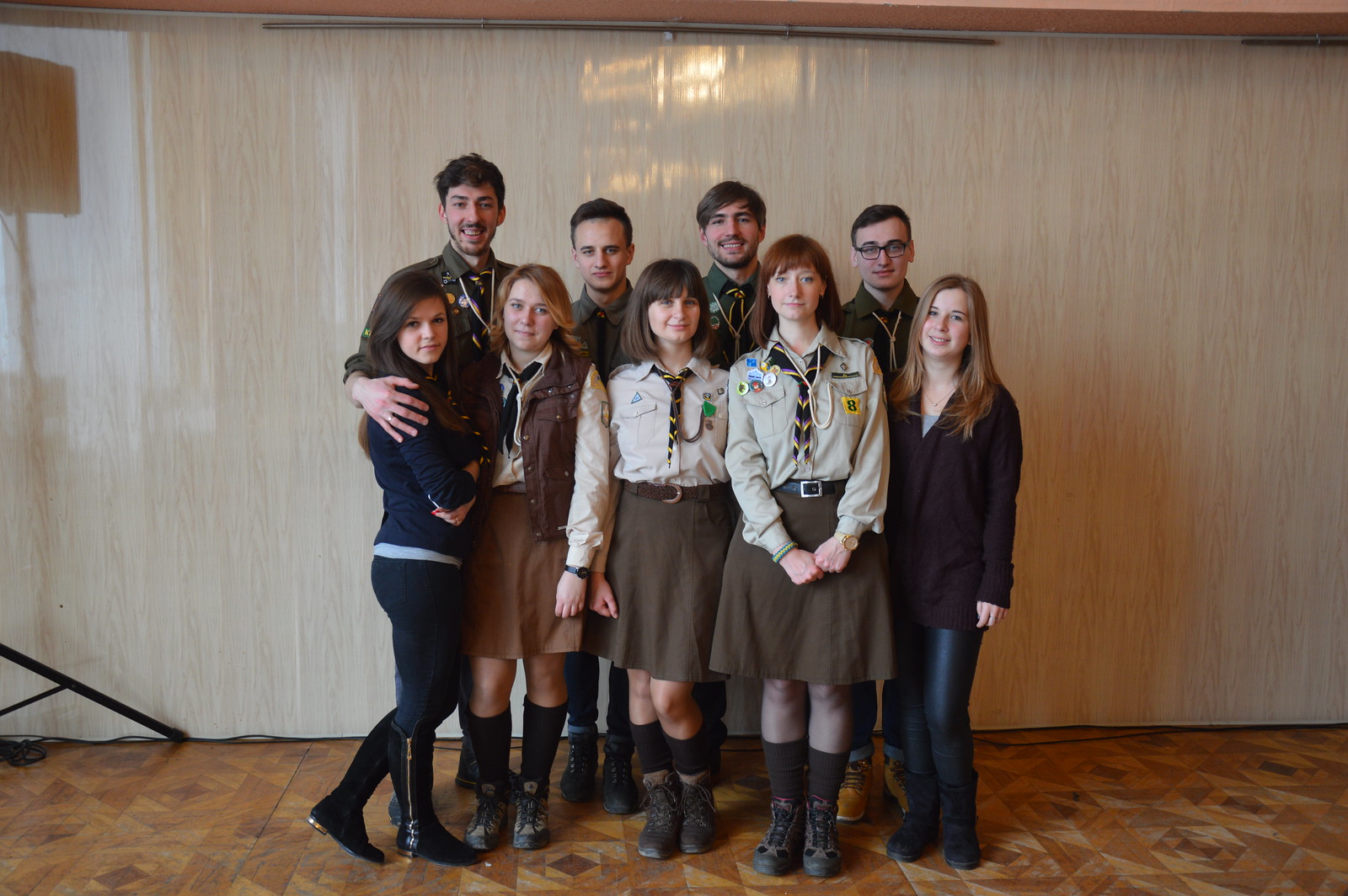This group photo showcases nine teenagers standing against a wood-colored wall. The front row consists of five girls, with two centrally positioned girls wearing matching tan collared long-sleeve shirts, reminiscent of Girl Scout uniforms, paired with skirts that fall just above their knees. The girl to their right dons a plain black long-sleeve shirt, tight black pants, and boots. On the left side, another girl is wearing dark blue leggings, black boots, and is partially turned inward. She is embraced by a man behind her. Another girl, second from the right, is dressed in a similar uniform but distinguishes herself with a brown vest over her attire. The backdrop is made of materials resembling vinyl siding, and the group stands on a light-tiled floor. The four boys in the back row, taller than the girls, appear to wear high-collared long-sleeve shirts that suggest they might also be uniforms, though they are obscured by the people in front. The boy on the far right wears glasses. The overall setting may include an old overhead projector in its rolled-up state.